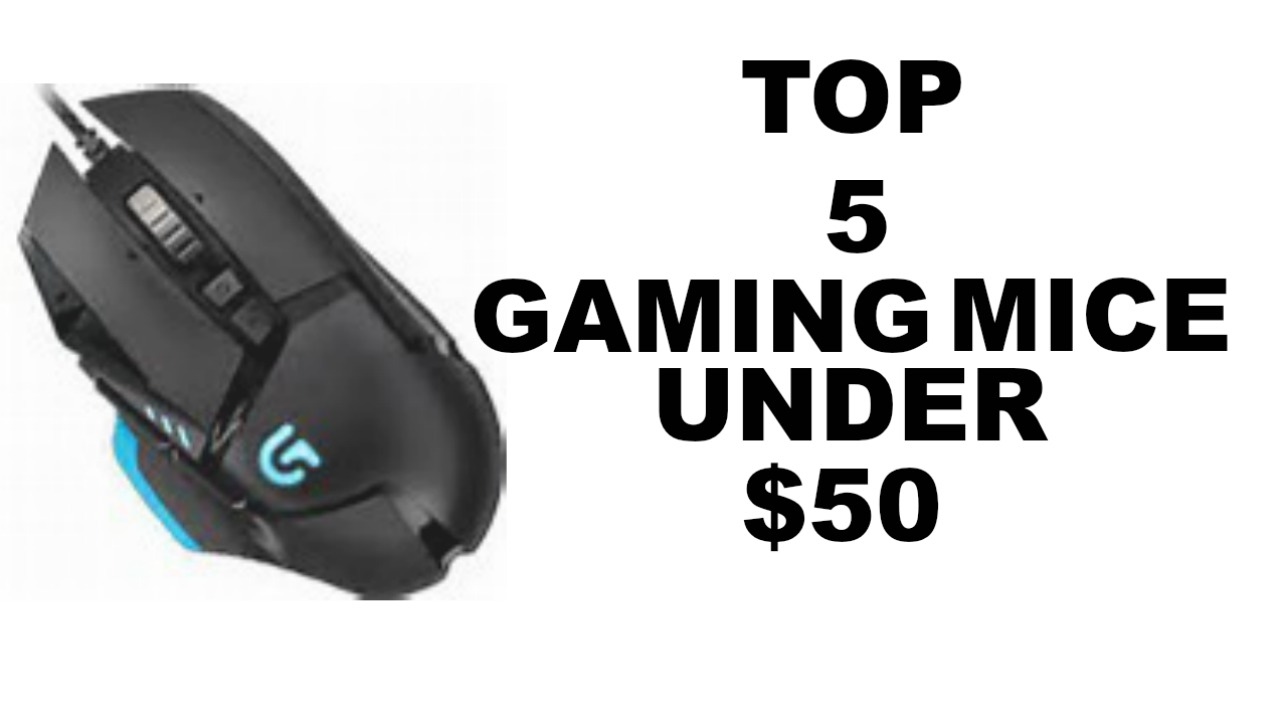**Caption:**

Featured prominently on the left side of the advertisement is a sleek, black gaming mouse with a unique design. The mouse showcases an all-black body with a distinctive scroll wheel occupying a significant portion of its middle section. A notable gap divides this scroll wheel, and just above the gap, a bold blue "G" logo—presumably representing the brand—stands out. Adding to its striking appearance, a blue line accents the side of the mouse, leading up to a cord that connects off-screen at the top. The entire advertisement is set against a clean, white background. On the right side, large black text reads, "Top 5 Gaming Mice Under $50," clearly indicating the purpose of the advertisement. The sophisticated design and branding suggest that this gaming mouse is part of a curated list of budget-friendly, high-performance gaming peripherals.